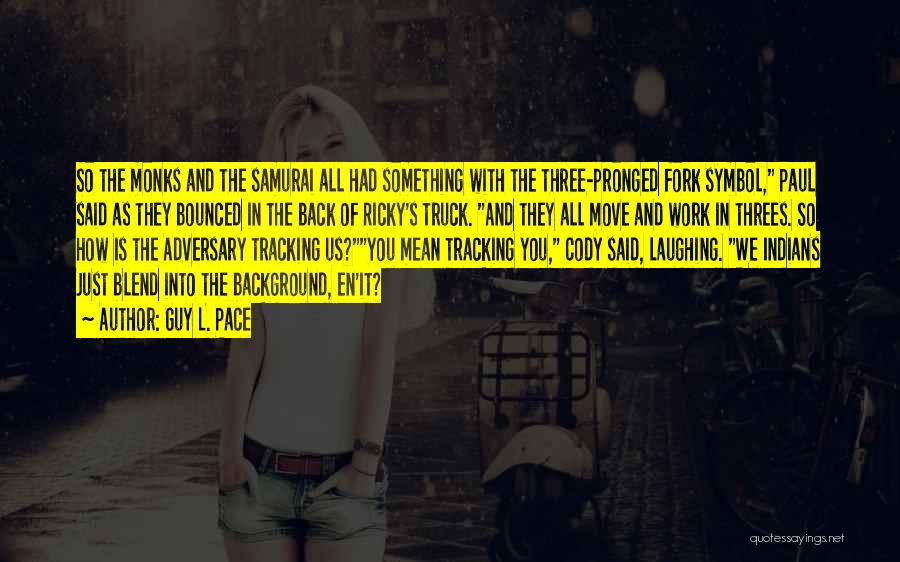In a predominantly black and white cityscape, a blonde woman stands confidently in a narrow alley, next to a motorized bike and a bike rack filled with bicycles. The urban backdrop is marked by buildings and possibly rainy or snowy conditions. She's dressed in a white sleeveless shirt, blue jeans, and a distinctive leather belt that may appear reddish. Her hands are tucked casually in her pockets, and although her face is partially obscured by text, she seems to be smiling. On her wrist, there appears to be a watch, bracelet, or possibly a tattoo. Superimposed over the image is a quote in capitalized, black sans-serif font highlighted with a yellow background. The quote, attributed to Guy L. Pace, reads: "So the monks and the samurai all had something with the three-pronged fork symbol, Paul said, as they bounced in the back of Ricky's truck and they all move and work in threes, so how is the adversary tracking us? You mean tracking you, Cody said, laughing. We Indians just blend into the background, innit?" The text "quoteessaythings.net" appears in white letters at the bottom of the image, adding a final touch to the composition's layered narrative and design.